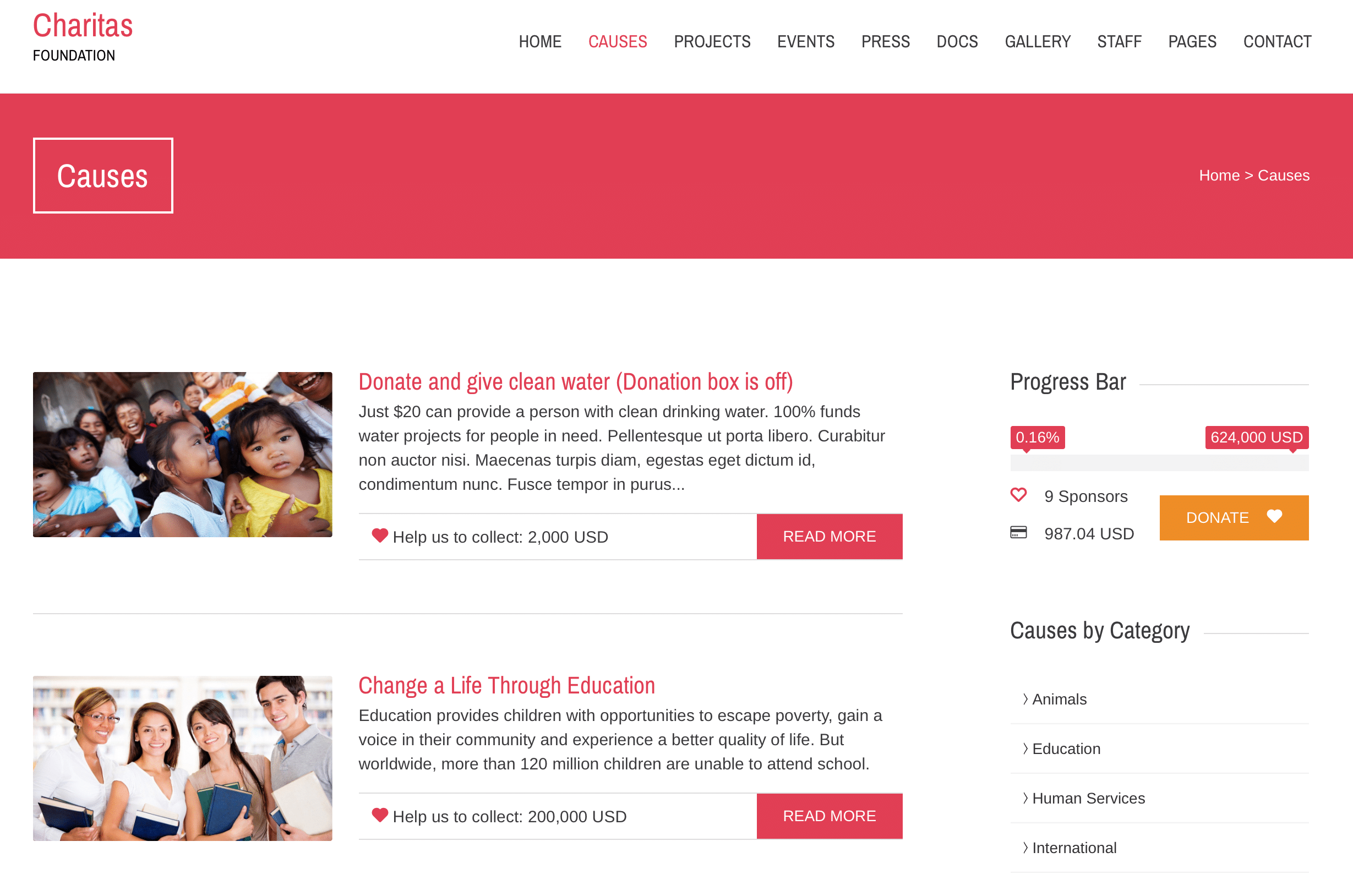This screenshot portrays the homepage of the Cheritas Foundation website. In the upper left-hand corner, the word "Cheritas" is displayed in light red text, resembling "Caritas" but with an 'H'. Just below, "Foundation" is written in black text, situated on a white banner that stretches across the top of the page. This banner also houses several clickable links, including 'Home', 'Causes', 'Projects', 'Events', 'Press', 'Docs', 'Gallery', 'Staff', 'Pages', and 'Contact'.

Beneath the white banner, a red banner appears, mostly empty except for a white-outlined box on the left-hand side, inside which "Causes" is written in white text – indicating the user has clicked on the 'Causes' tab. 

Further down, two articles are stacked vertically. Each article features a thumbnail image on the left. The first photo depicts a group of children and is titled "Donate and Give Clean Water" in red text. An excerpt from the article is displayed below the title in black text, followed by a red 'Read More' button. The second article shows an image of four young adults and carries the title "Change Your Life Through Education" with similar excerpts and navigation options.